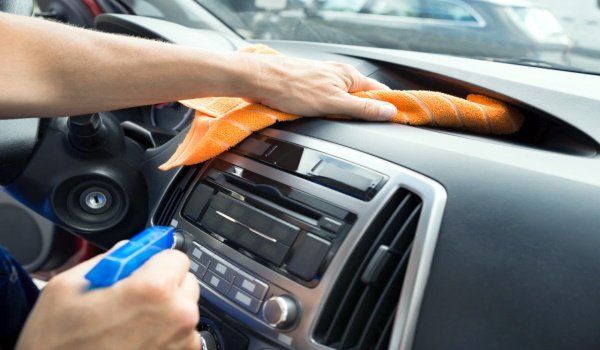The image depicts a close-up of the interior of a car, showing a granite gray dashboard with silver trims. Two hands are visible in the frame, engaged in cleaning the car's center console. The right hand holds a blue spray bottle, while the left hand brandishes an orange terry cloth rag, wiping down the gray and shiny surface. The console features various components: a silver ignition keyhole, a radio with black air vents on either side, multiple buttons, and knobs, as well as a CD player with an ejection button. In the background, a slightly dirty windshield is visible with sunlight shining through, revealing a glimpse of a few other cars outside.